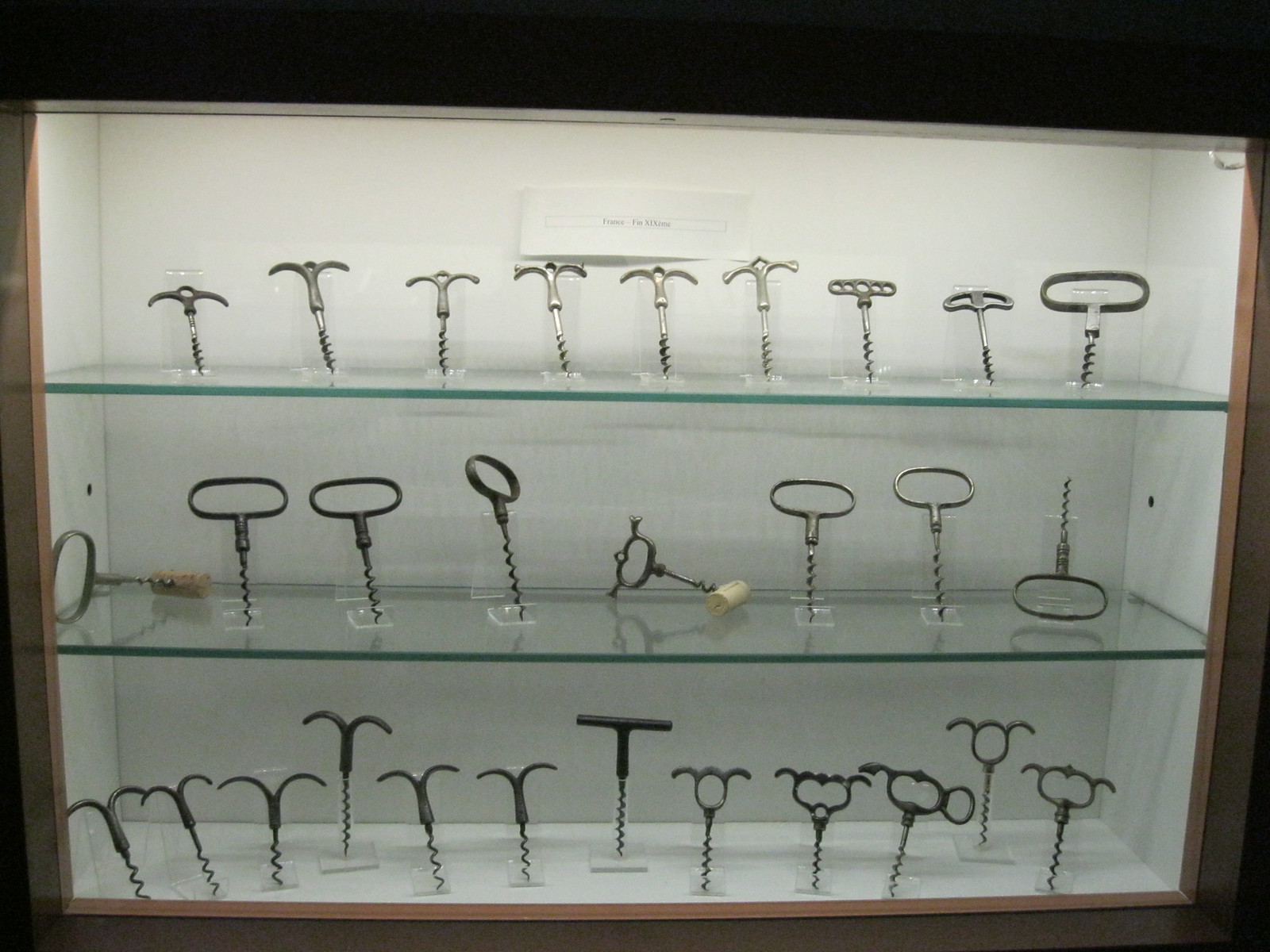The photograph is a close-up, color image of a glass-fronted display case with wooden edging, presented in a landscape orientation. The lighting within the display case illuminates the various corkscrews inside, although the outer edges of the image, particularly the top part, are underexposed and in shadow. The display case is angled slightly from the top left to the bottom right in the frame.

Inside the case, there are three equally spaced glass shelves showcasing an array of corkscrews, displayed both vertically and horizontally. The corkscrews appear to be of different styles and from different time periods, ranging from newer, metal-loop designs to older, dark iron pieces. In total, there are nine corkscrews on the top shelf, eight on the middle shelf—two of which have corks attached—and several more on the bottom shelf. Some corkscrews are standing upright in transparent perspex stands, while others are lying flat, with a mix in the orientation of handles and screw tips.

The lighting within the display case enhances the intricate details of the corkscrews, hinting at their historical and possibly antique nature. There is also a piece of paper with tiny, unreadable text behind the corkscrews, suggesting a museum exhibit.